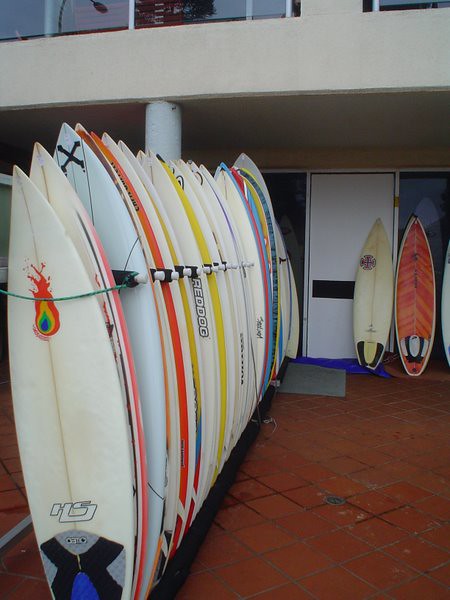This photograph captures a colorful and detailed scene of approximately 20 to 30 surfboards standing vertically in a row, secured together by a green wire and separated by black plastic spacers. The surfboards, with colors ranging from white, blue, yellow, red, and orange, are positioned on a reddish-orange terracotta tiled floor, which features a center drain suggestive of a bathing or shower area. The surfboards are supported by a plastic rack and are predominantly aligned on the left side of the image, with one surfboard showcasing a flame motif against a cream background in the foreground. Behind these surfboards stands a beige stone building with visible elements that include windows, a white door, and a pillar. Additionally, two surfboards lean against the wall and door, one white and one reddish, framed by what appears to be the lower part of a hotel or apartment building. The detailed composition and vibrant colors of the surfboards create an engaging and dynamic image.